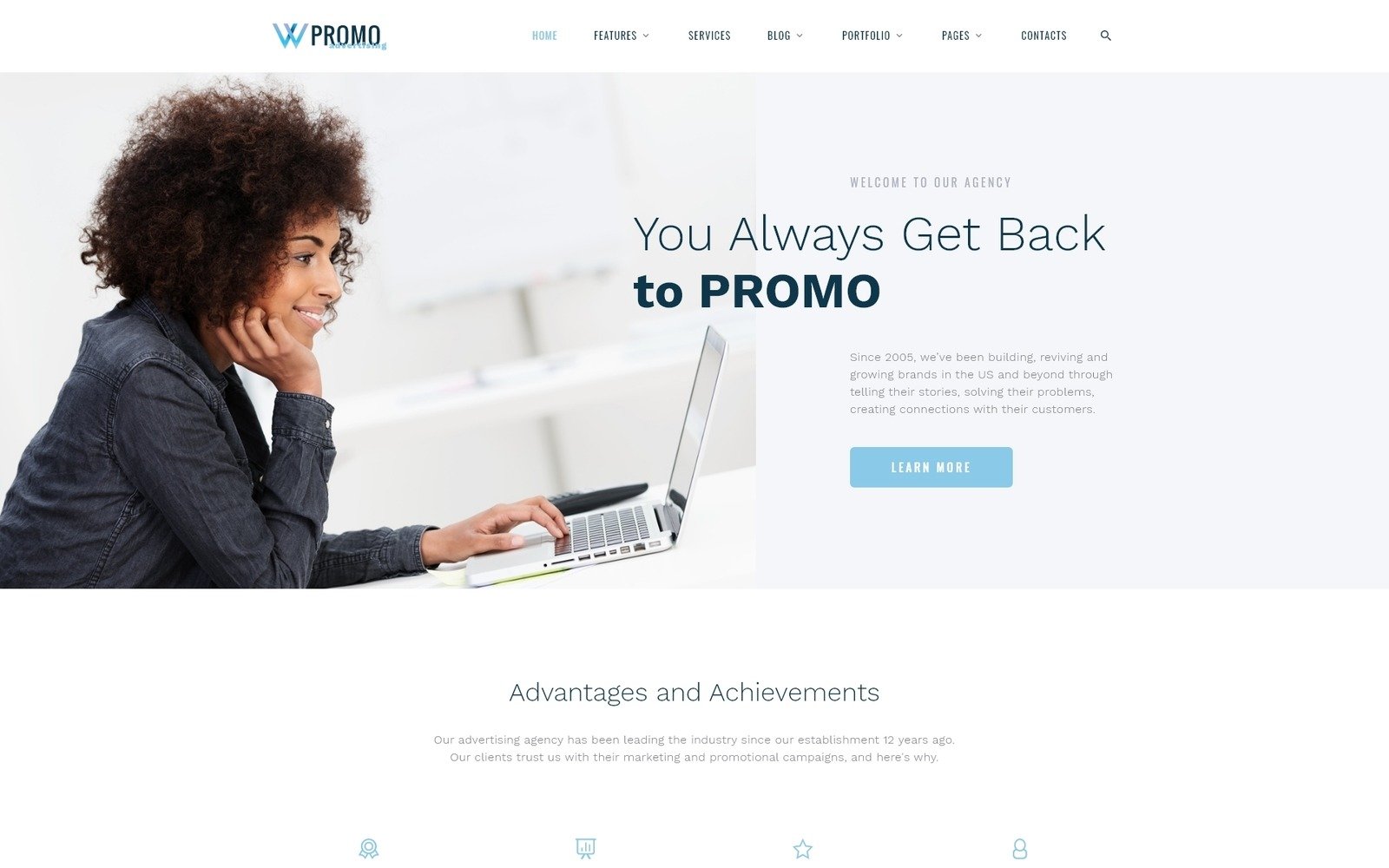This promotional image from a company called "Promo" prominently features the company's name in the upper left corner. Centrally displayed is a large, blue "W." Across the top, the navigation menu includes options in black text: "Features," "Blog," "Portfolio," "Pages," and "Contacts," accompanied by a search icon. The central image showcases a smiling Black woman using a laptop, with her right hand thoughtfully cupping her chin as she engages with the screen. The image is overlaid with a welcoming message: "Welcome to the Agency," followed by a brief introductory paragraph and a blue "Learn More" button. Below this, there are sections labeled "Advantages," "Achievements," along with a brief description, though the text is difficult to read. At the bottom, several icons are visible, but only a star is distinguishable, as the rest are faint. The background is very light, featuring subtle shelving behind the woman, contributing to the overall light and airy aesthetic of the image.